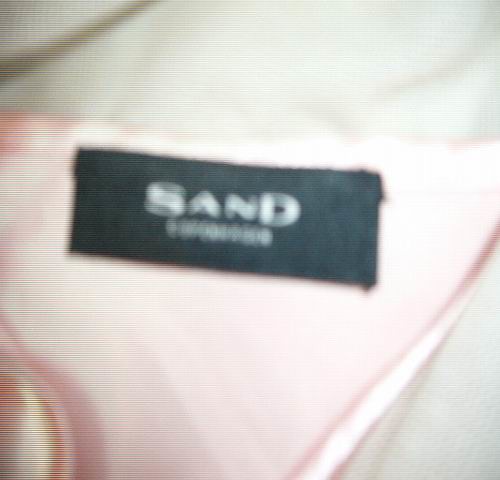The image depicts a very blurry up-close shot of a pink shirt or cloth folded atop a beige sheet, with another layer of white fabric partially visible underneath. Dominating the center of the composition, there is a dark rectangular label with the large white text "sand," accompanied by an unreadable, smaller white text below it. A faint black strip appears to the top left of this label. The photograph's overall low clarity makes it difficult to discern finer details, while a shadow or a darker pink wrinkle is noticeable in the bottom left corner, likely contributing to the obscurity.